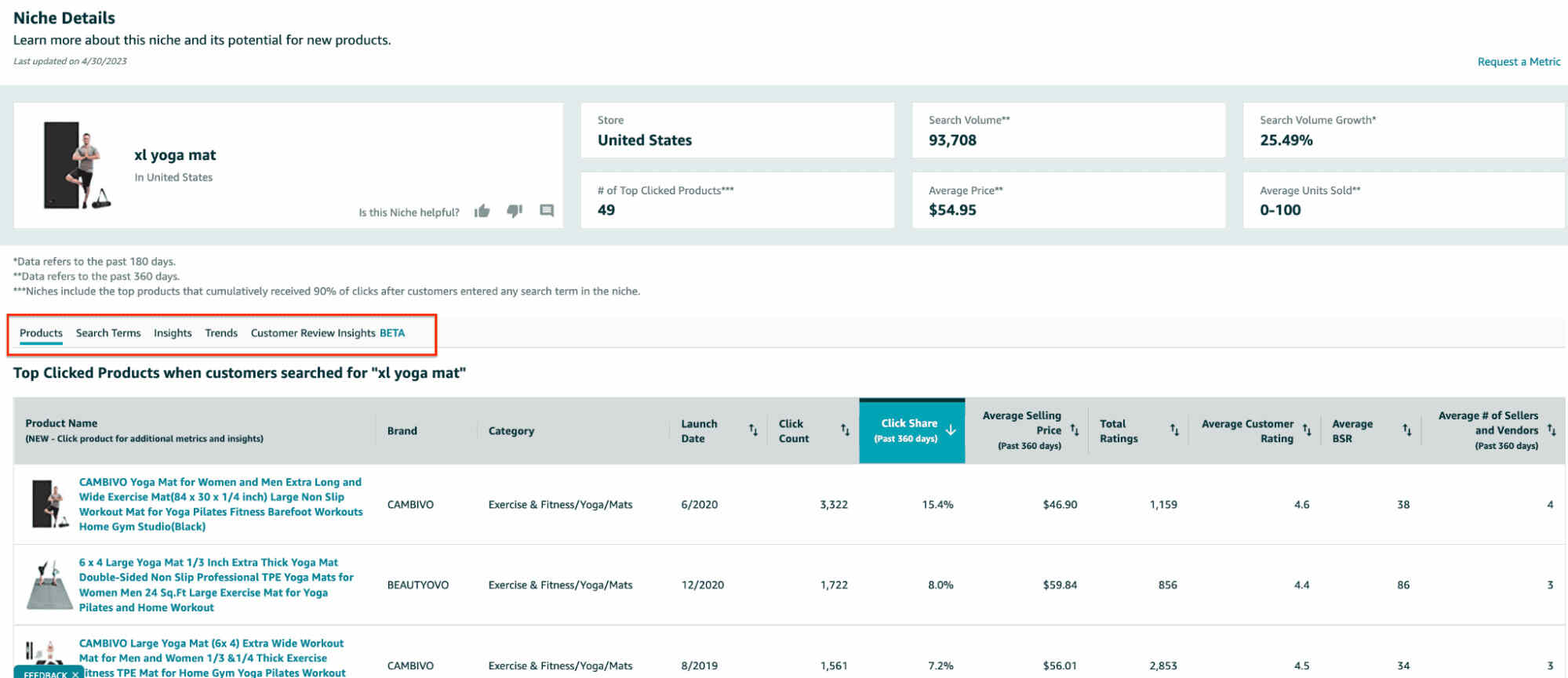Detailed Caption:

A comprehensive dashboard presents niche-specific details on the left panel, prompting users to "Learn more about this niche and potential for new products," with an update timestamped to April 30, 2023. Directly below, the niche focus is highlighted as "Extra Large Yoga Mat in United States," alongside interactive feedback options including a thumbs-up, thumbs-down, and a comment section.

The statistics for the United States market indicate that there are 49 top-clicked products related to this niche, with a substantial search volume of 93,708. The average price of these yoga mats is $54.95, and the search volume growth is recorded at 25.49%. Average units sold are categorized within the range of 0-100. Above this data, the blue label "Quest a metric" is prominently displayed.

Additional information clarifies that the data reflects observations from the past 100 and 360 days, marked by one asterisk for 180 days, two for 360 days, and three asterisks explaining that niches include the top products that collectively receive 90% of clicks from customers entering any related search term.

Below these insights, navigation tabs labeled "Products," "Search Terms," "Insights," "Trends," "Customer Reviews," and "Insights Beta" are outlined within a red rectangle, indicating the different sections available for further exploration. The overall layout suggests an instructional purpose, showcasing how users can analyze top-clicked products when customers search for "Extra Large Yoga Mat."